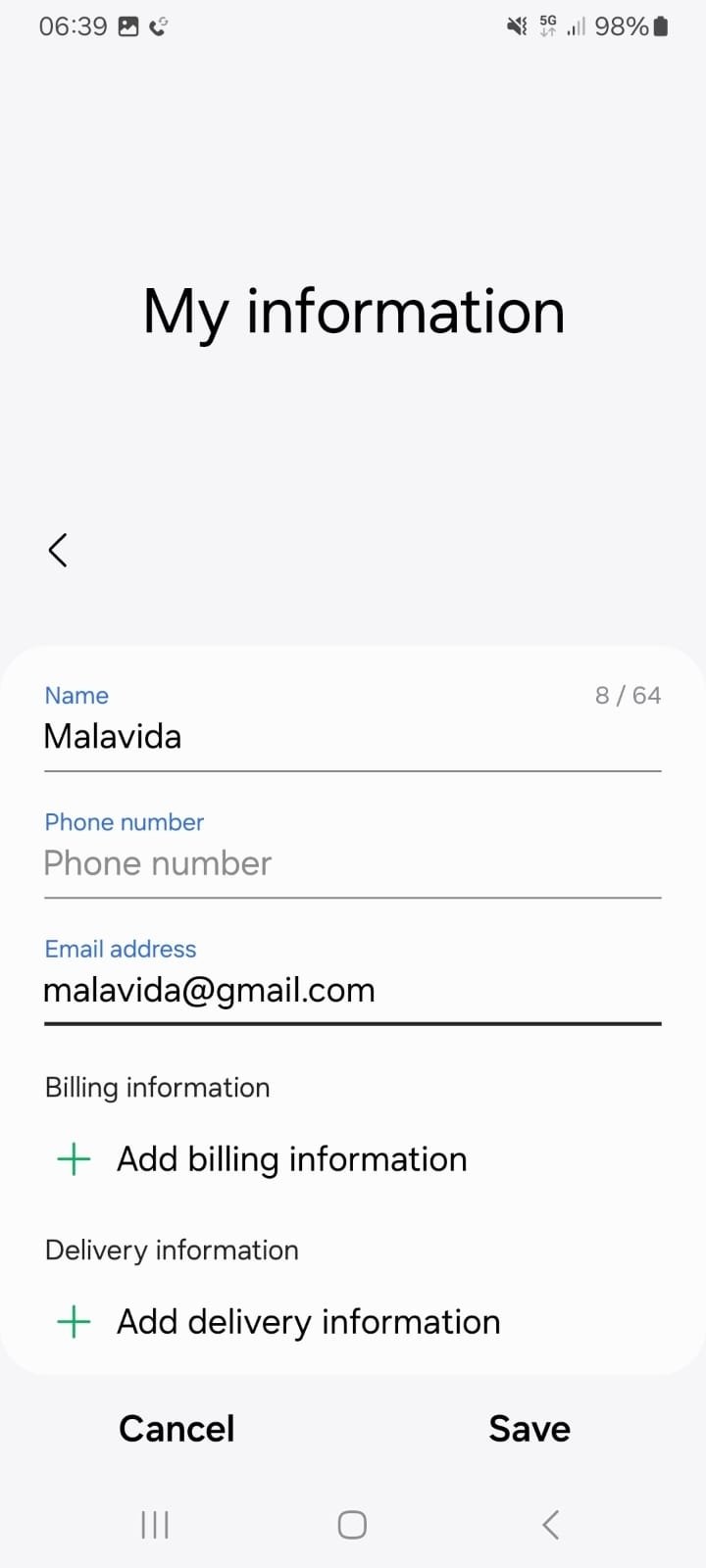This screenshot captures an Android smartphone screen while the user is filling in information on a website form. The interface displays the time as 6:39 in the top left corner, alongside several notification icons. The top right corner shows three crucial status indicators: a muted speaker symbol, a 5G network icon, and a battery level at 98%.

Directly below these indicators, the screen's backdrop is a clean, light shade—either white or light gray. Centered at the top of the screen in bold black text is the title "My Information." To the left of this header is a back arrow icon.

The main portion of the screenshot reveals a form with multiple fields. The form's background is white, and the fields' labels are in blue text, marked as "Name," "Phone Number," and "Email Address." The "Name" field is populated with "Malavita," the "Phone Number" field is blank, while the "Email Address" field shows "malavita@gmail.com."

Below these fields, there are sections for adding "Billing Information" and "Delivery Information." Each section features a green plus symbol and the prompt to add the relevant details, but both sections remain unfilled.

At the bottom of the screen, two prominent buttons are displayed: "Cancel" on the left and "Save" on the right. Underneath these buttons are the phone's navigational icons for general app or screen navigation: three horizontal gray lines on the bottom left, a gray square in the bottom center, and a gray back arrow on the bottom right.